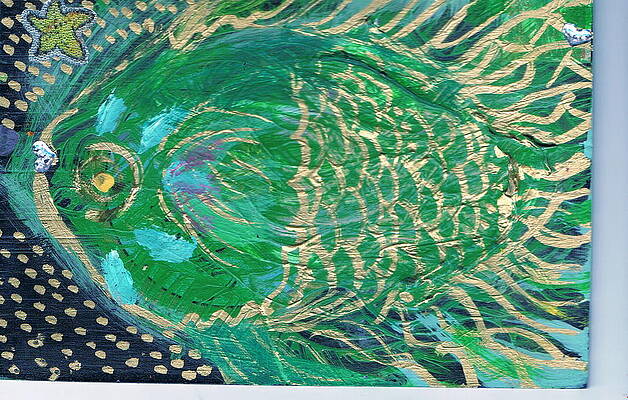The image showcases a stylized, impressionistic painting of a large green fish rendered in what appears to be oil paint, hanging on a whitish-blue wall. The fish's eye is strikingly yellow, and its body is adorned with golden scales and outlined with gold paint, which also accentuates its flowing fins. The thick, textured swirls of green paint, including rich forest green and teal, add depth and character to the fish. Surrounding it, the background is predominantly black and features numerous golden dots, creating a visually engaging contrast. In the upper left corner of the painting, a yellow starfish outlined in both black and white floats above the fish. Additionally, touches of blue and turquoise, along with some yellow and light blue elements, can be seen throughout the painting, enhancing its vibrant and dynamic composition.